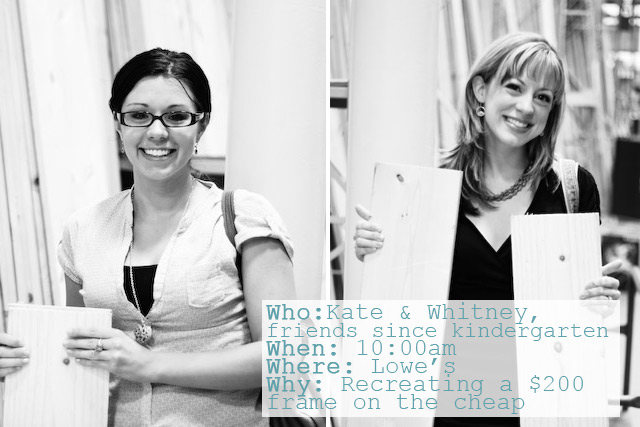This black and white photograph captures two smiling women, identified as Kate and Whitney, lifelong friends since kindergarten, as revealed by superimposed text. Both women are holding small pieces of wood in their hands, likely part of a project mentioned in the text, "Recreating a $200 frame on the cheap." Kate, on the left, has her black hair tied back, wears glasses, and is dressed in a black tank top beneath a white short-sleeve shirt. She accessorizes with a low-hanging necklace, a ring, and a purse slung over her shoulder. Whitney, on the right, has blonde hair flowing past her shoulders, wears a black dress, and adorns herself with a necklace, earrings, and a backpack. They are standing in front of an indistinct background, possibly walls or buildings, and the time stamp "10 a.m. Where? Lowe's" indicates the setting of their project. Both women project joy and camaraderie through their shared expression.